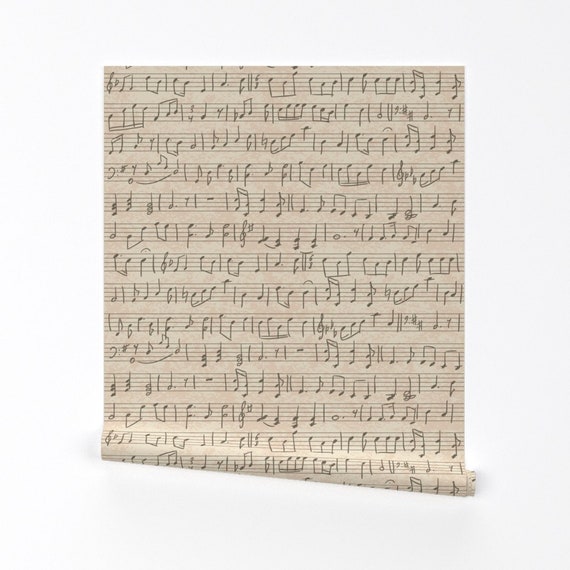The image depicts a detailed musical score handwritten on a brown scroll of paper, creating an elegant downward slope at the bottom where the paper curls up. The sheet is densely filled with musical notes arranged across ten lines, divided into staves that run from left to right. Notable details include the presence of a G clef in the top left corner, indicating it is a treble clef score. The entire composition is set against a plain white background, emphasizing the rich, intricate patterns of the black musical notes.